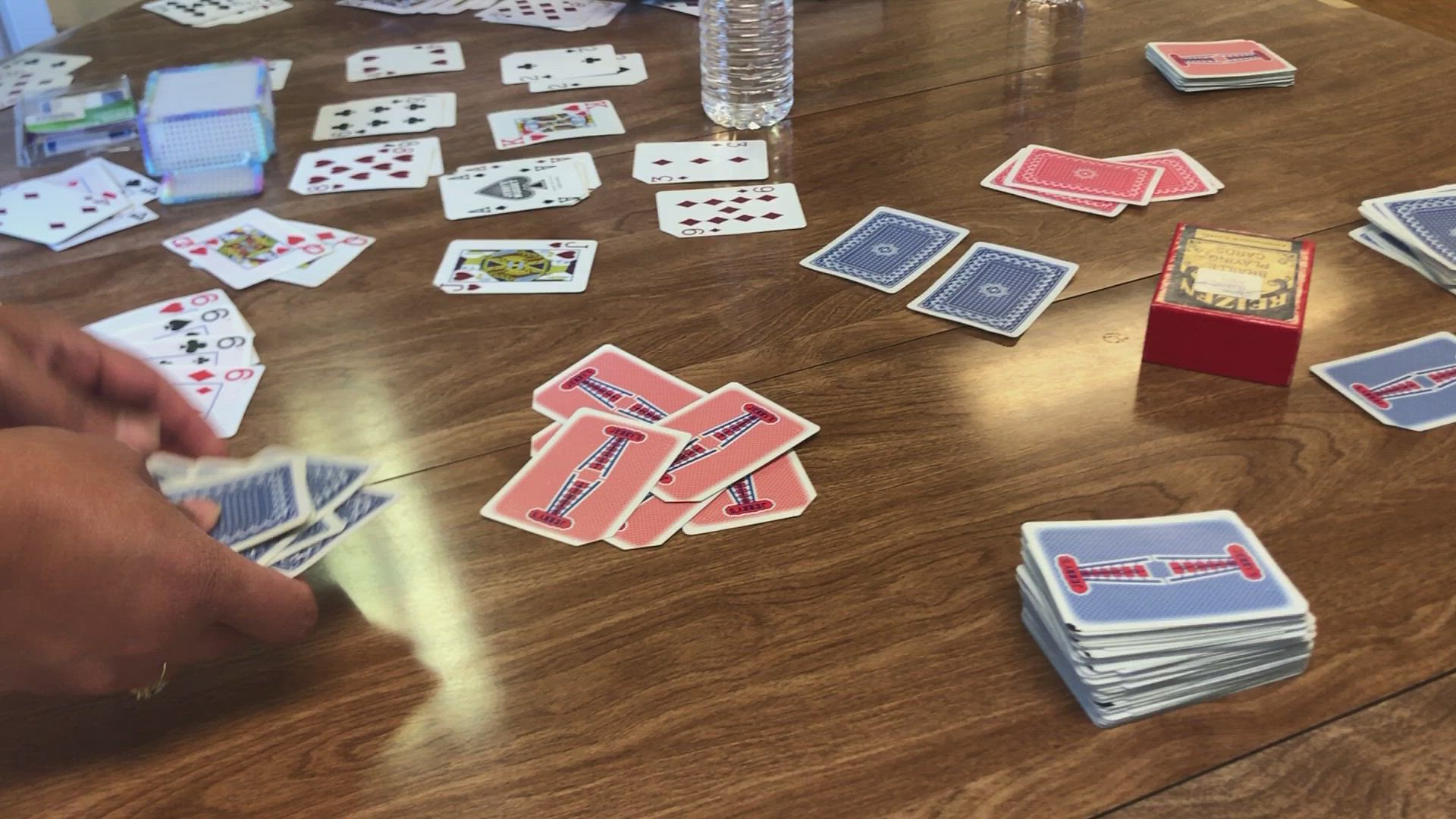The color photograph features a beautifully polished, brown hardwood table covered with an array of playing cards. In the center of the table, numerous cards are stacked and spread out, showcasing their light blue backs adorned with a red bar design. Toward the upper right-hand corner, a deck box is visible with red sides and a golden top featuring intricate designs, though slightly out of focus.

In the lower left-hand corner, a pair of large hands, likely belonging to a medium dark-skinned Black man, holds several cards face down. Scattered across the table, particularly in the upper left-hand corner, some cards lie face up, revealing the king of spades, the ace of spades, the queen of hearts, and another indistinct face card. The presence of these cards suggests an ongoing game among multiple players. At the very top center of the image, the base of a water bottle is visible, completing the lively and detailed scene.